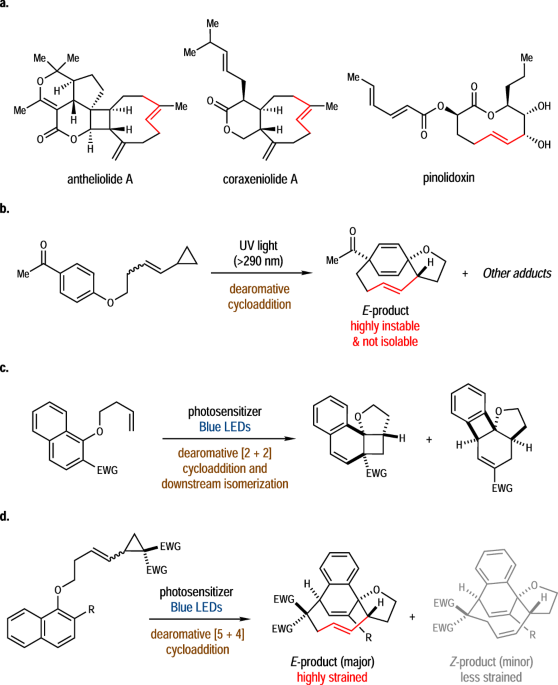The image presents a detailed diagram of various chemical molecules displayed on a white background, divided into four labeled sections: A, B, C, and D. In section A, molecules labeled as antheliod (or anthelialide), chora-hexionalide, and pinolidoxin are depicted with black molecular structures, some highlighted in red. Sections B and D feature molecules undergoing processes indicated by arrows: section B notes the involvement of UV light (>290 nm) and "DRO-mattive cycloaddition," while both sections B and D include annotations for "photosynthesizer blue LEDs," leading to the formation of new molecular structures. In section C, a molecule with the acronym EWG is shown splitting into two different molecules due to photosensitization by blue LEDs. Different lines, including solid, double, and red lines, connect the hexagonal and other shapes, with text in various colors, including brown, red, and blue, annotating the diagram.